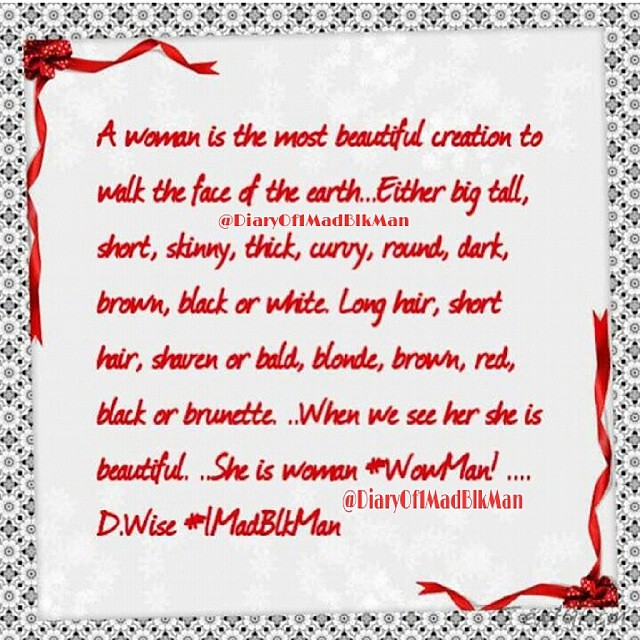This image depicts a graphic quote framed by a black and white floral border. Both the upper left and lower right corners feature red ribbons with white polka dots tied into bows, with ribbons extending vertically and horizontally in an L shape. The centerpiece of the graphic is a quote, written in red handwritten script, which reads: "A woman is the most beautiful creation to walk the face of the earth. Either big, tall, short, skinny, thick, curvy, round, dark, brown, black, or white. Long hair, short hair, shaven or bald, blonde, brown, red, black, or brunette. When we see her, she is beautiful. She is woman. #WowMan!" Additionally, the text includes "D wise," "#IMadBLKMan," and the handle "@DiaryOfOneMadBlkMan" in smaller font, suggesting the author's social media presence. This detailed design resembles a note card or social media graphic celebrating the beauty and diversity of women.